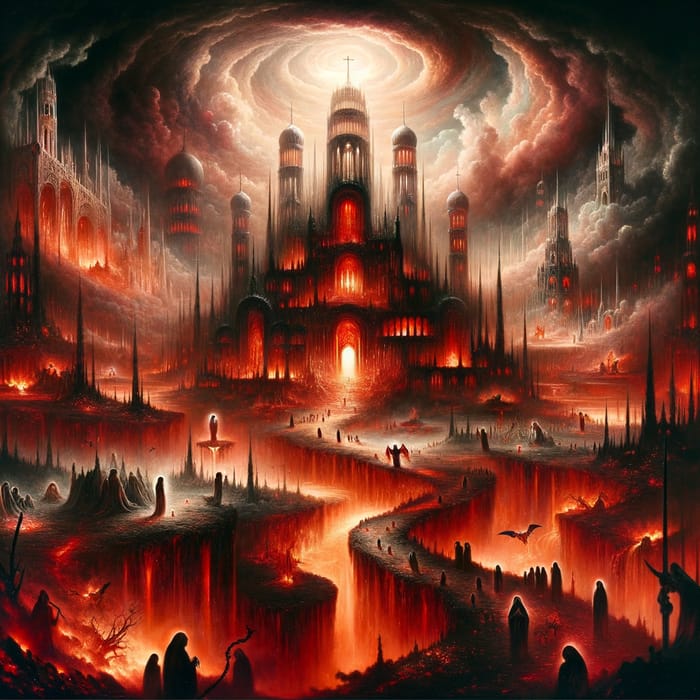The image depicts a dark and foreboding painting, likely set in a medieval or fantasy universe, evoking a sense of dread and chaos. Dominating the center is a major castle, featuring five towers adorned with crosses, illuminated from above by a beam of sunlight piercing through swirling, spiraling clouds that create an otherworldly atmosphere. The painting's dark undertones are accentuated by the extensive use of black paint, interspersed with fiery red and orange hues suggestive of lava, which surround the lone path leading to the central castle, giving the impression of a hellish landscape. Minor castles and structures pepper the background, each similarly engulfed in the ominous glow of the lava-like substance that fills the bottom of the composition. Small, black-drawn characters traverse the narrow, elevated pathways, some seemingly trapped by the surrounding sea of lava, while bats ominously fly overhead. The scene appears to be a nightmarish vision or representation of hell, complete with smoke swirling upwards, highlighting the castle and its architecture in a ghostly luminescence, creating an overall terrifying and chaotic tableau.